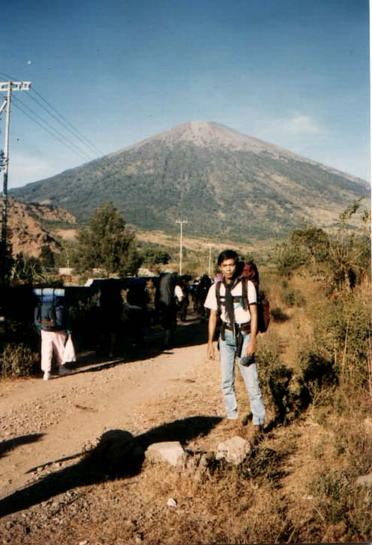In the photograph, a young man, possibly a teenager, stands on a dirt trail with a large volcanic mountain looming in the background. The trail winds through a dry, beige-colored landscape dotted with sparse shrubs and scrubby bushes. The young man, framed against a deep blue sky with minimal clouds, gazes directly into the camera. He is dressed for hiking in a white t-shirt, light-colored jeans, and brown boots, with a large red backpack secured to his back by black straps crossing his chest and stomach. Attached to his belt is a camp knife. The setting sun casts long shadows, indicating the late hour of the day. In the mid-ground, a group of hikers with backpacks walk the dirt path towards the gray, rocky mountain, which tapers to a light, jagged peak, indicative of its volcanic nature. Telephone poles and utility lines stretch off into the distance, suggesting the area is not completely remote. The vintage quality of the photograph gives it a slightly dingy, older feel, adding to the sense of adventure and timelessness captured in the image.